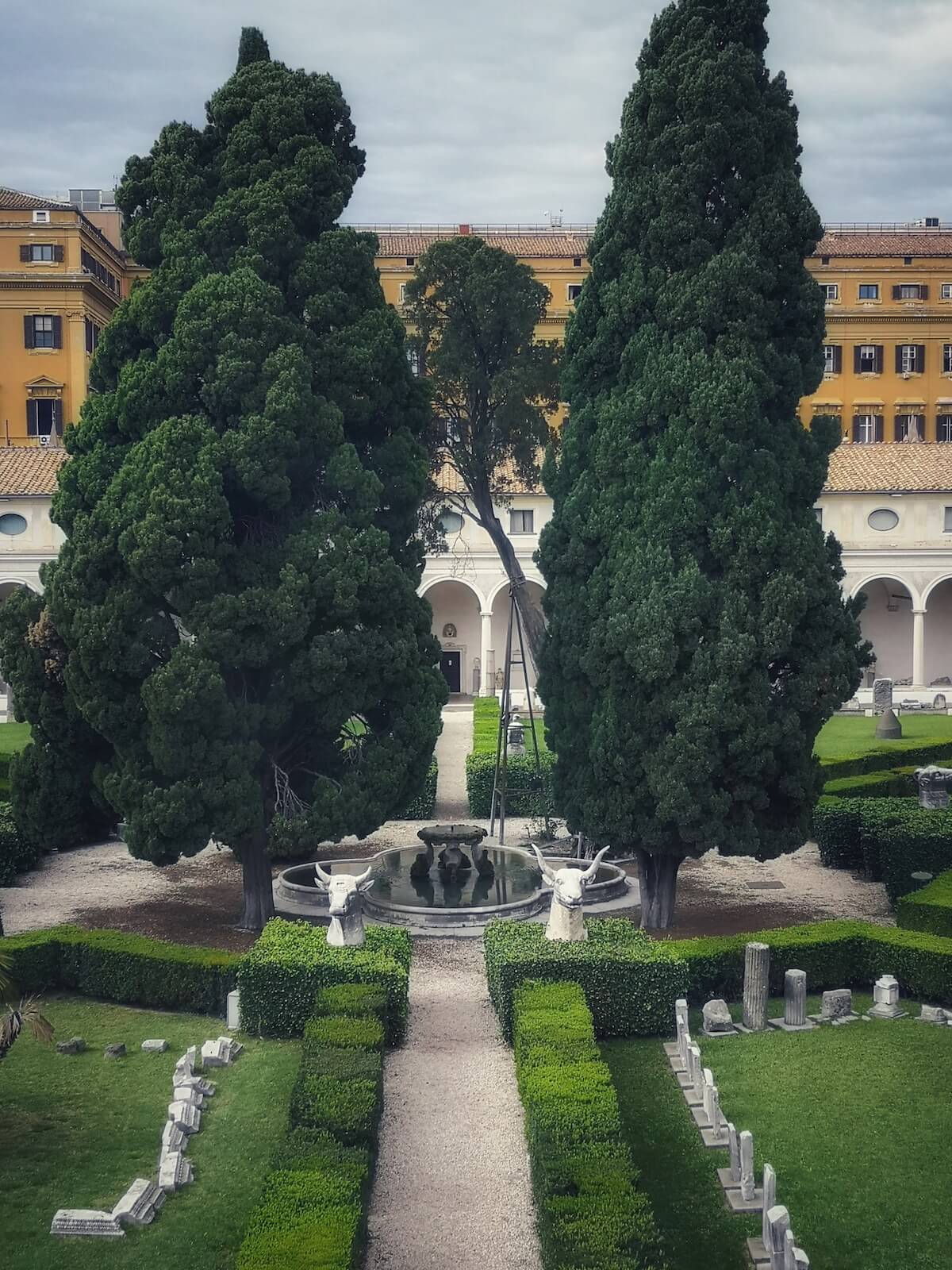In this detailed photo of an English garden, an elegant courtyard unfolds before a grand, historic villa. The villa, characterized by its dual-tone facade of tan on the upper portion and white on the lower, boasts a series of impressive arched pillars. Positioned prominently in front of this stately building is a large, circular water fountain, flanked symmetrically by tall cedar trees. The fountain design is unique, featuring two semicircular extensions on either side, creating a striking centerpiece.

In the foreground, meticulously clipped square shrubs, reminiscent of a maze, add to the structured beauty of the garden. Atop these shrubs, there are two large stone statues of carved cow heads, strategically placed to enhance the visual appeal. One cow head sits on the left side, and the other on the right, both positioned just before the fountain.

A pristine white pathway runs through the center of the garden, leading directly to the fountain. This pathway is bordered by patches of lush grass interspersed with scattered white statues, adding a touch of elegance to the scene. The garden paths, radiating out from the central fountain area, guide visitors through the greenery and towards the villa. The sky overhead is overcast, casting a gray hue over the entire scene and providing a dramatic backdrop to this picturesque garden.